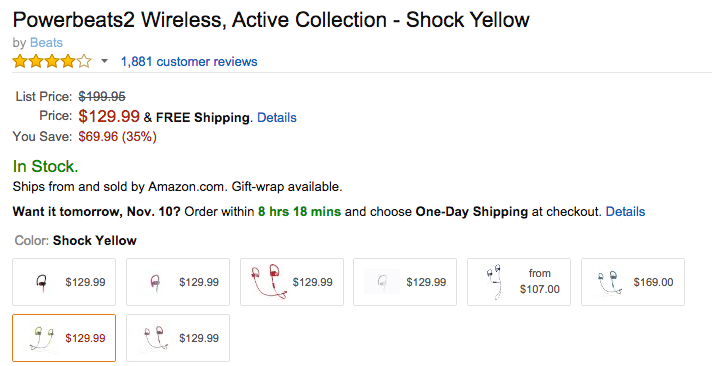This image is taken from an Amazon.com review page for the Power Beats 2 Wireless Active Collection in Dash Shock Yellow. The page prominently displays a mixed review summary with four out of five stars, where four stars are colored yellow and one star is white. Beneath this, it notes there are 1,881 customer reviews, highlighted in blue print. The product's list price was originally $199.96, now discounted to $129.99, marked in red print. Additionally, there's an indication that free shipping is available, detailed in black text beside a "Details" link in small blue print. Highlighting the discount, it also mentions the buyer saves $69.96 (35% off). The stock status is highlighted in green print, stating the product is "In Stock," and it's further mentioned in black text that the item "Ships from and sold by Amazon.com, gift wrap available." Lastly, there's an option to receive the item by the next day, November 10th, if the order is placed within 8 hours and 18 minutes.